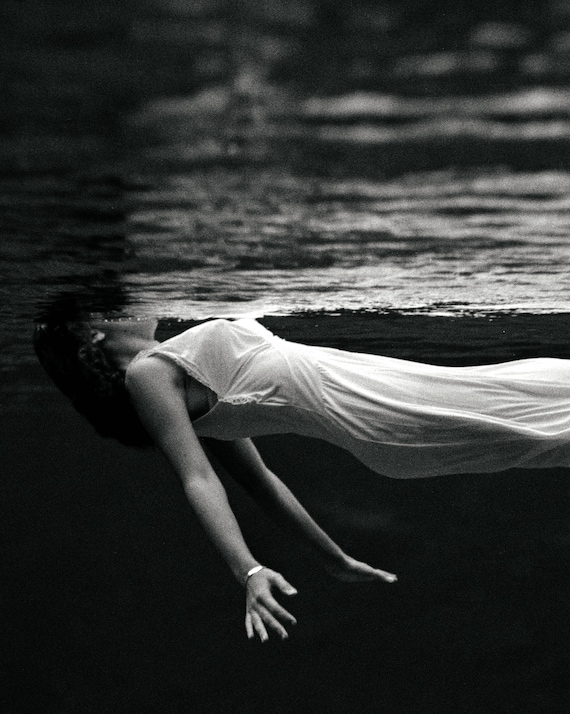This black-and-white photograph captures a woman floating horizontally just beneath the water's surface, with her face breaking through the top of the water, obscuring it. Her arms drift downward, and her body extends from the top of her head to her knees, which are cut off by the edge of the image. She is clad in a long, white, flowy dress that clings to her form due to the water, making the dress slightly see-through and revealing she is wearing underwear beneath it. Her dark, medium-to-long hair fans out in the water. A metal bracelet, likely gold, adorns her left wrist. The surface of the water features light ripples, adding texture to the top half of the image. The rest of the scene is devoid of any additional objects or text, focusing solely on the serene, underwater moment.